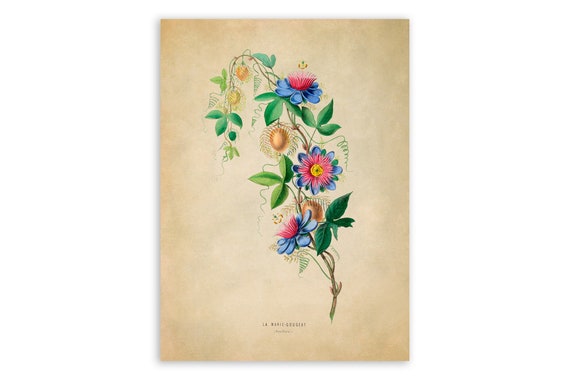This image is a vintage-style drawing of a floral arrangement on a coffee-stained, cream-colored paper with discolored edges. The artwork features a simple, centered bouquet of flowers and plants, extending from the top to the bottom of the page. The flowers include blue petals with pink centers, as well as pink and white round blossoms with yellow centers. The plant exhibits green leaves that extend from the stem, with additional artistic vines and leaves that seem to be an interpretation rather than realistic. There's also a yellow-green fruit resembling a kumquat. Though there is text underneath the plant, it is too small to read, adding to the overall vintage and artistic feel of the drawing.